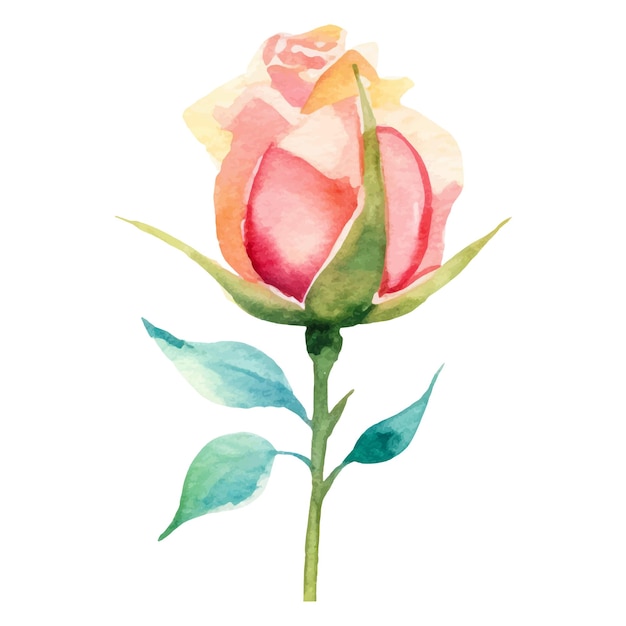This image is a detailed watercolor painting of a flower that could be a rose or a tulip, characterized by its pastel shades and abstract appearance. The flower’s bud, which is just about to bloom, showcases a harmonious blend of soft pinks, dark reds, light oranges, pale yellows, creamy whites, and peachy tones, giving it a delicate and almost ethereal quality. The painting captures the essence of the flower with slightly runny watercolors, adding to its abstract, dreamy feel. The stem is depicted in a solid, pastel green with a few thorns and supports three bluish-green leaves, exhibiting aquatic hues from dark aqua to light aqua and green. The entire composition stands against a pristine white background, emphasizing the flower's pastel colors and airy presence without any framing or additional context. This depiction evokes a sense of tranquility and beauty, making it a very pleasant and visually appealing piece.